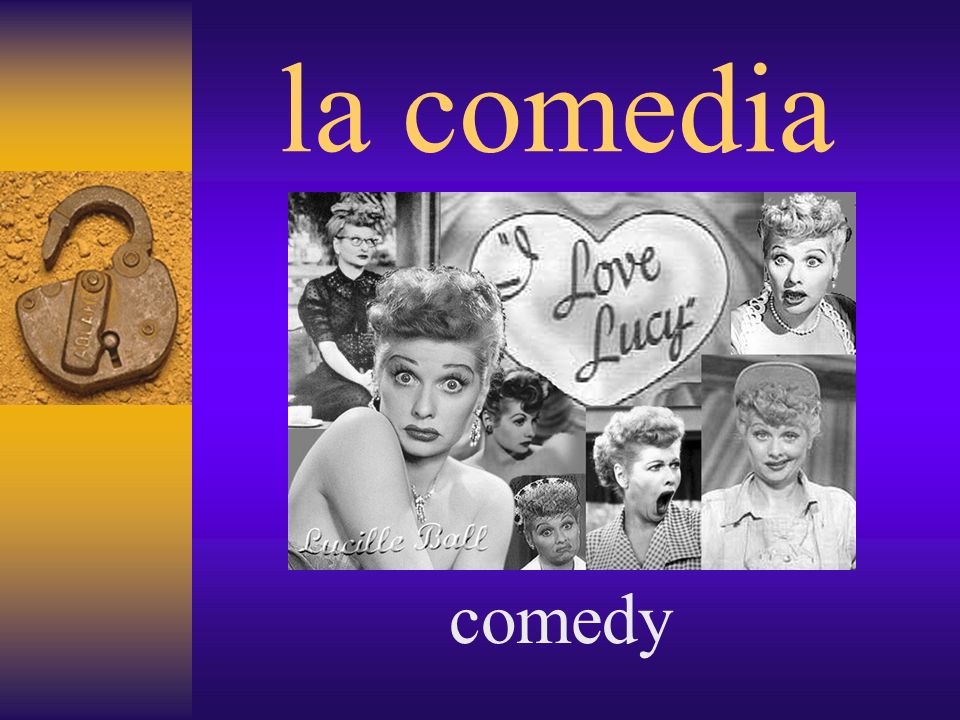This detailed colored print media piece celebrates the classic TV show "I Love Lucy." Dominating the design are seven black-and-white images of Lucille Ball, capturing her in various iconic expressions and moments from the show. At the very center of these images is the show's well-known heart logo with the text "I Love Lucy" inside. The top section of the piece features a blue gradient background with the text "La Comedia" in lowercase yellow letters, while at the bottom, it reads "Comedy" in lowercase white letters. 

Adding a peculiar element, the left-hand section of the print is an orange gradient background, which distinctively contrasts the blue. This section becomes even more intriguing with the insertion of a very old-fashioned, open brass padlock in the center, resembling those operated with a skeleton key. Despite its unclear connection to the TV show, the padlock adds a historical and mysterious touch to the overall design. Throughout the print, the name "Lucille Ball" is prominently featured, highlighting the legendary actress associated with the memorable "I Love Lucy" series.